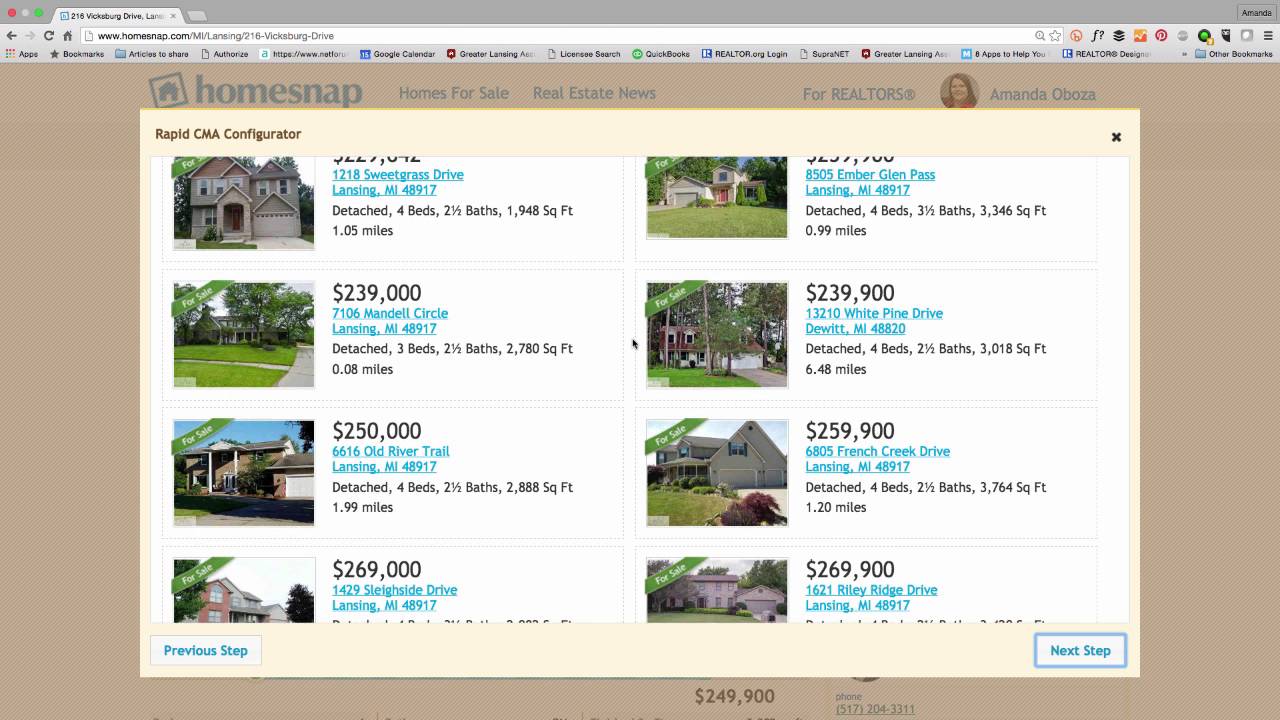This image depicts a homes-for-sale website with the top-left corner featuring the logo and name "HomeSnap." To the right, in gray text, it reads, "Homes for Sale, Real Estate News, 4 Realtors." A circular profile picture of Amanda Aboza, a dark-haired woman with pale skin, is also visible.

Below this, in the middle-left section, there is an image of a house with multiple pointed roofs, located at 1218 Sweetgrass Drive, Lansing, Michigan, 48917. The house is a detached property featuring 4 bedrooms, 2.5 bathrooms, and 1948 square feet of living space. The house's proximity is 1.05 miles from a reference point.

Next to this, there is another house that appears longer but smaller compared to the first. This house is situated at 8505 Ember Glen Pass, Lansing, Michigan, 48917. It also is a detached home, boasting 4 bedrooms, 3.5 bathrooms, and a more spacious 3346 square feet, located 0.99 miles from a reference point. 

To the left, there's a listing for a house priced at $239,000, located at 7106 Mandel Circle, Lansing, Michigan, 48917. 

On the right side, another house is pictured amid abundant trees. It is listed for $239,900 and located at 13210 White Pine Drive, DeWitt, Michigan, 48820. This house features 4 bedrooms, 2.5 bathrooms, and 3018 square feet of living space, situated 6.48 miles from a reference point.

Further down, there is an image of a brown house listed for $250,000, located at 6616 Old River Trail, Lansing, Michigan.